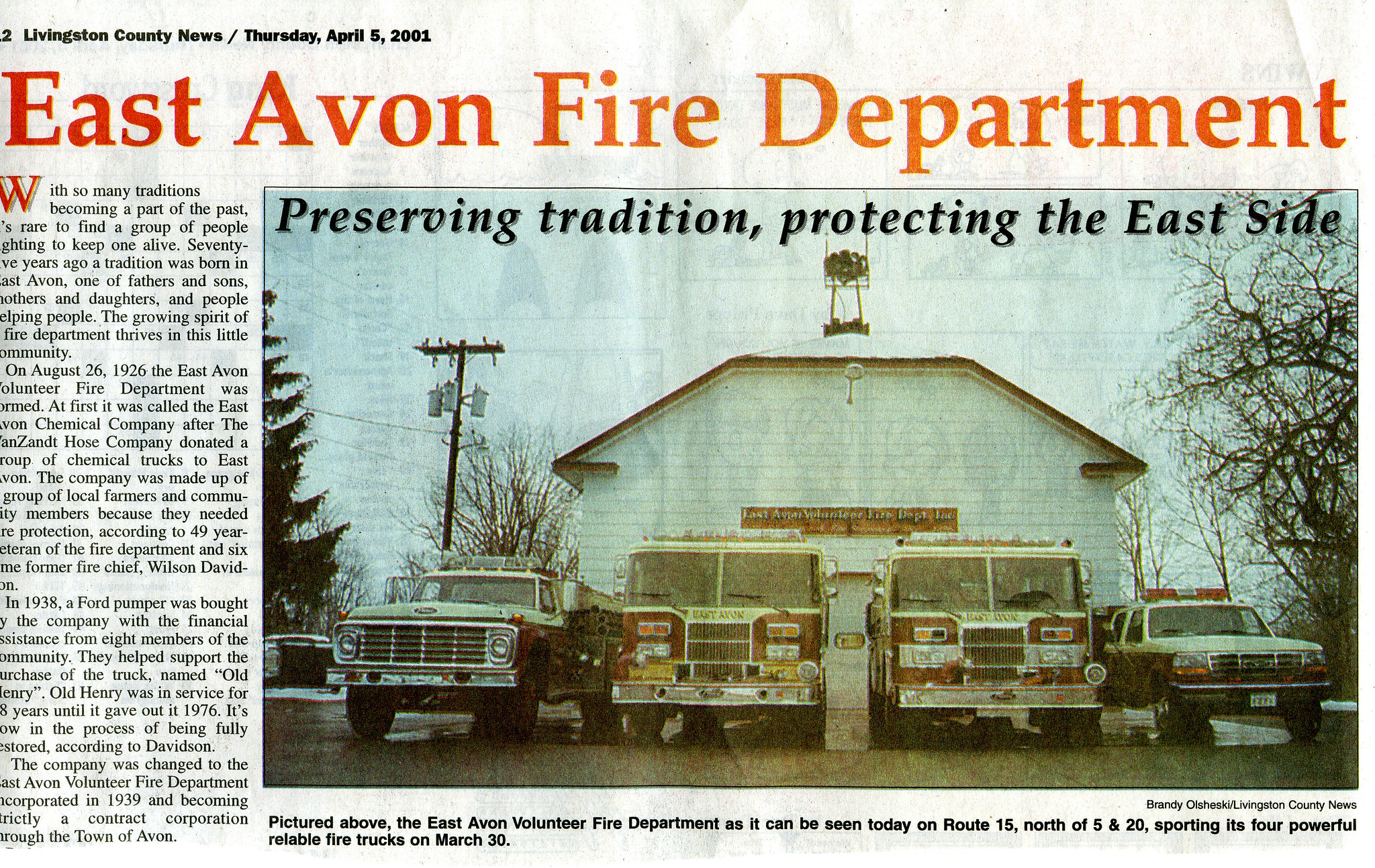This image is a photograph of a newspaper clipping from the Livingston County News, dated Thursday, April 5, 2001. Large, bold red letters at the top of the image announce "East Avon Fire Department." The headline beneath it reads, "Preserving Tradition, Protecting the East Side." The photograph within the clipping depicts the East Avon Volunteer Fire Department as it stood on Route 15 north of routes 5 and 20, showcasing four emergency vehicles—two central fire engines and two additional emergency trucks on either side. The fire station is a white building with a flat roof, topped by a siren and possibly an antenna or tower. The setting is complemented by trees, including a barren tree on the right and a pine tree on the left, under an overcast sky. A telephone pole is visible on the left of the image. The caption under the picture reads, "Pictured above, the East Avon Volunteer Fire Department as it can be seen today on Route 15 north of 5 and 20, sporting its four powerful, reliable fire trucks on March 30." The adjacent article starts with a decorative red "W" and discusses the efforts to maintain tradition within the fire department.